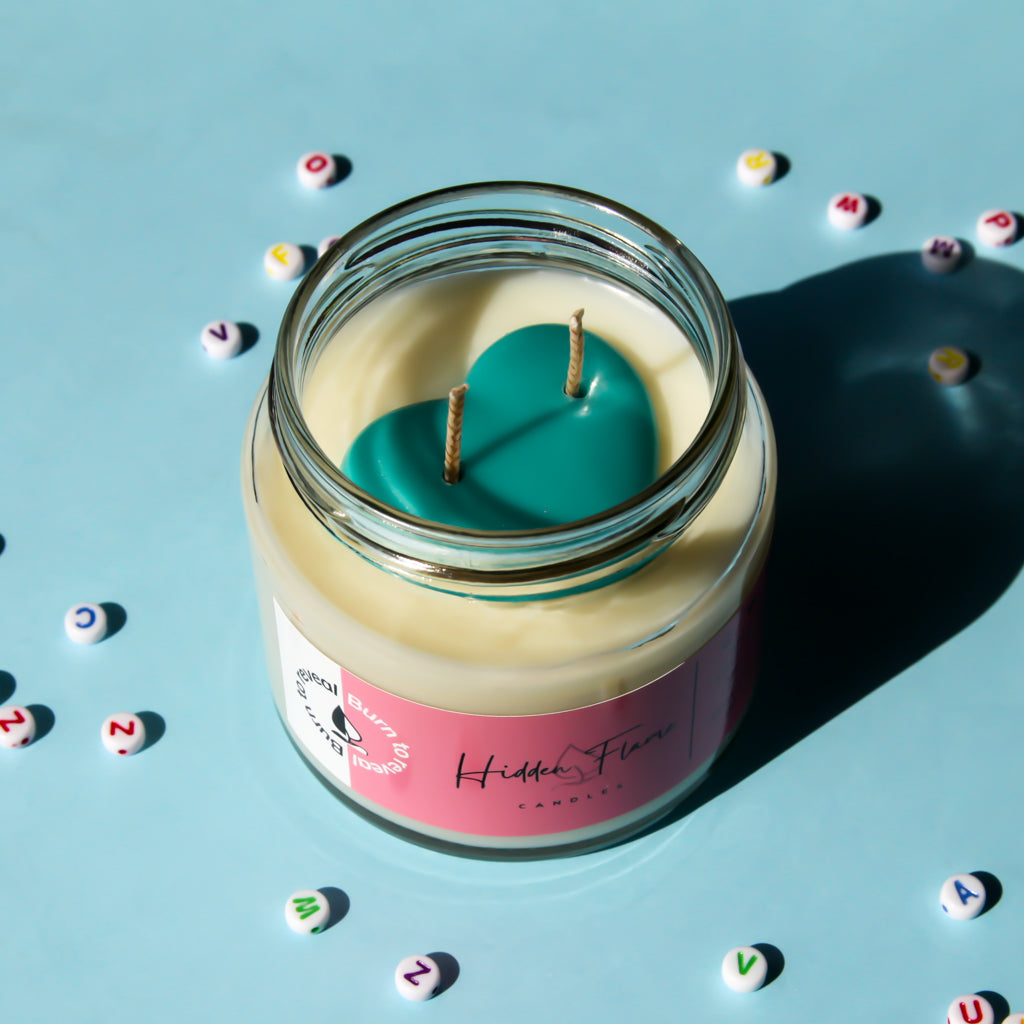A square image showcases a glass jar containing a dual-wicked candle. The main body of the candle is cream-colored, featuring a heart-shaped segment in an off-blue, blue-green hue. Adorning the front of the jar is a pink label with a black section that includes white lettering. The label reads "Hidden Flame Candles" and incorporates a leaf emblem hidden within the flames. On the far left of the label, there are additional white areas featuring black text that partially reads "Burn To," though the rest of the text is indistinguishable. The jar rests on a blue surface, which is sprinkled with small, white circular dots that have various letters and colors. The scene is subtly enhanced by the shadow of the candle cast behind it.